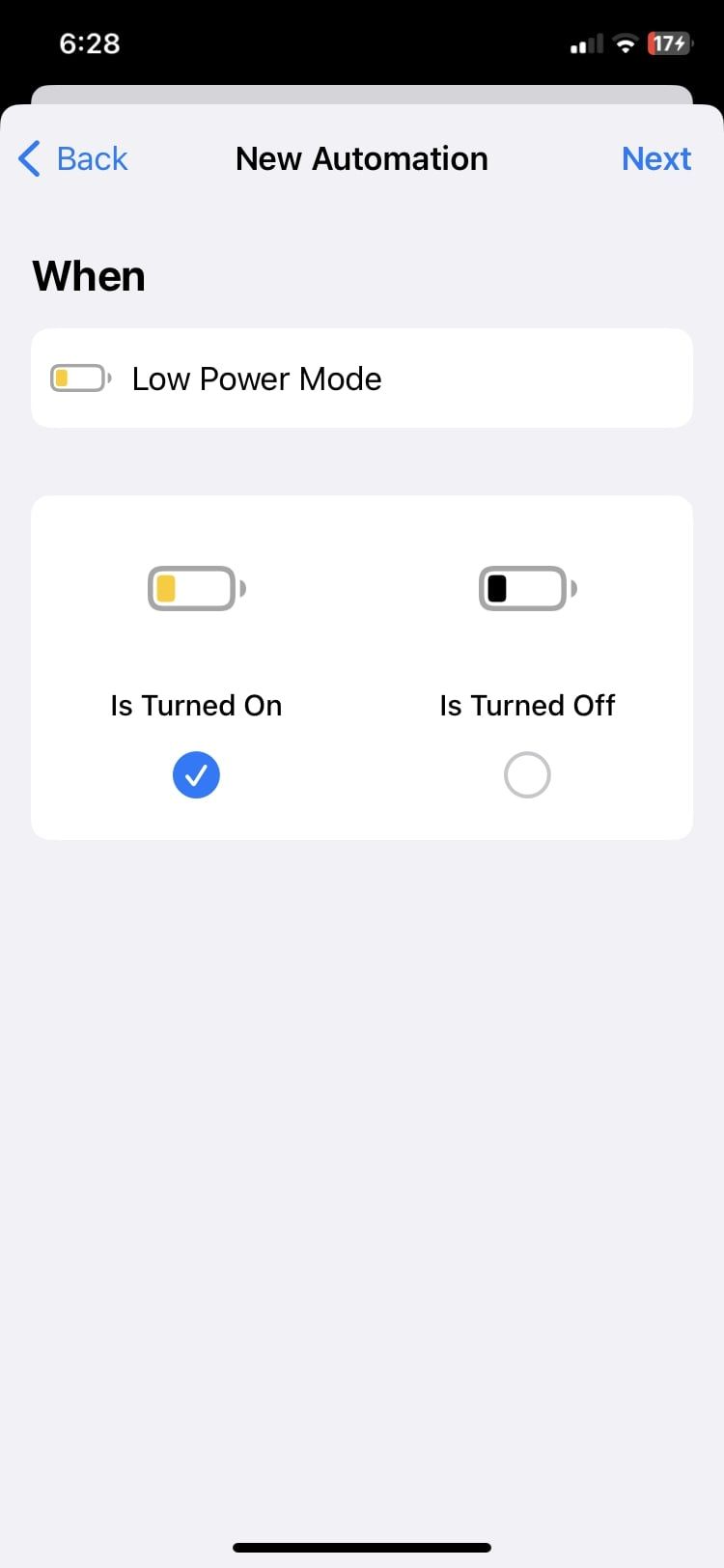The image displays an iPhone screen with a typical layout. At the top, there's a black status bar reminiscent of a phone's home screen, showing the time as 6:28 on the left, signal bars, WiFi signal, and a battery level of 17%, indicated by a red icon.

Beneath this status bar is the main screen of an app, showcasing a user interface for setting up a new automation. At the top of this interface, there is a blue "Back" button on the left, the word "Next" on the right, and centered between them is the title "New Automation" in black text.

The content of the screen is focused on creating an automation based on battery status. Under the heading "When", there is a white box displaying a selected condition, "Low Power Mode", with a yellow battery icon to the left and the text "Low Power Mode" in black. Below this, another white box outlines two conditions: "Is Turned On" with a checked box and a yellow battery icon, and "Is Turned Off" with an unchecked box and a black battery icon.

At the very bottom of the screen, there is a simple black line, indicating the end of the visible content. The overall screen is dedicated to setting up a specific automation within the app, likely related to battery management.